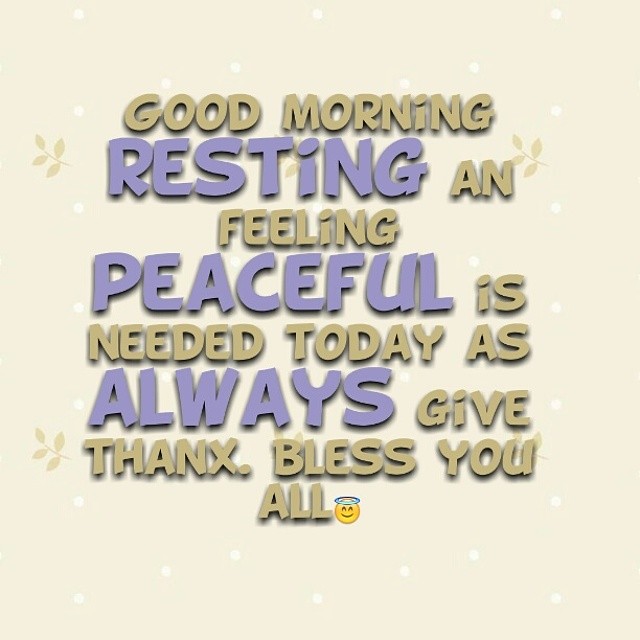This digitally drawn square-shaped e-card features a soothing cream background adorned with small white dots and delicate light brown branches with golden leaves, creating an autumnal vibe. The prominent text, neatly printed in uppercase letters, reads: "Good Morning. Resting and feeling peaceful is needed today. As always, give thanks, bless you all." Some words like "resting," "peaceful," and "always" appear in eye-catching periwinkle shades, while the rest of the text is in a beige or golden tan hue, giving a harmonious contrast. The words seem to have a slight 3D effect with subtle shadows. At the bottom of the card, a yellow smiling emoji with a blue halo adds a cheerful touch, emphasizing the inspirational theme.